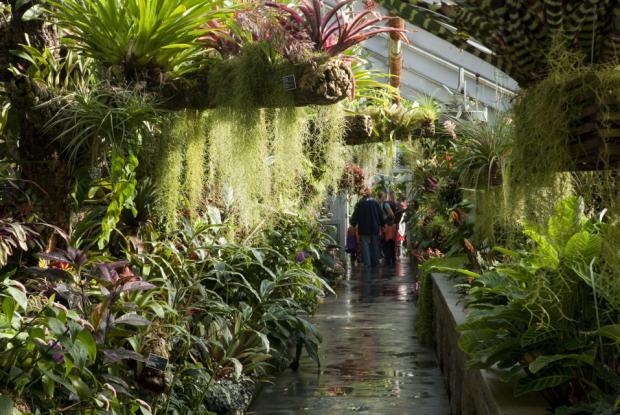In a lush indoor atrium filled with tropical foliage, a slightly damp and possibly slippery pathway runs through the center of the scene, leading towards a partially obscured white building in the background. The walkway, lined with a mix of vibrant green shrubs, tropical plants, and some purple and reddish flowers, creates a picturesque route amidst the greenery. Among the diverse plant life, there are large leaves, flowering plants, and hanging Spanish moss adding to the jungle-like ambiance. On one side of the pathway, there's an elevated stone garden, and on the other, flowering leafy plants at ground level. Prominent wooden beams and unique siding structures frame the space, enhancing the indoor garden feel. A group of people, including a lady and a man in blue coats and jeans, a little child in an orange shirt and black pants, and possibly another child in a purple shirt, walk down the path, their backs turned towards the viewer as they head towards the building. A weathered wooden pole and some beams run along the walkway, contributing to the natural aesthetic of the atrium.